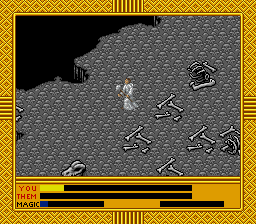This is a detailed screenshot from a game, framed by a yellow border adorned with small diamonds in varying shades of yellow. This border is intricately designed with a series of lines running along its top, bottom, right, and left edges. Inside the yellow frame, there is a smaller text box displaying the words "You," "Them," and "Magic." The word "You" features a piece of yellow, "Them" is entirely in black, and "Magic" is in blue. In the upper left-hand corner of the screenshot, there is a black abyss set against a gray background. A character dressed in white appears to be in motion within the scene. Trailing behind this character are numerous bones, which resemble those of an animal rather than a human.